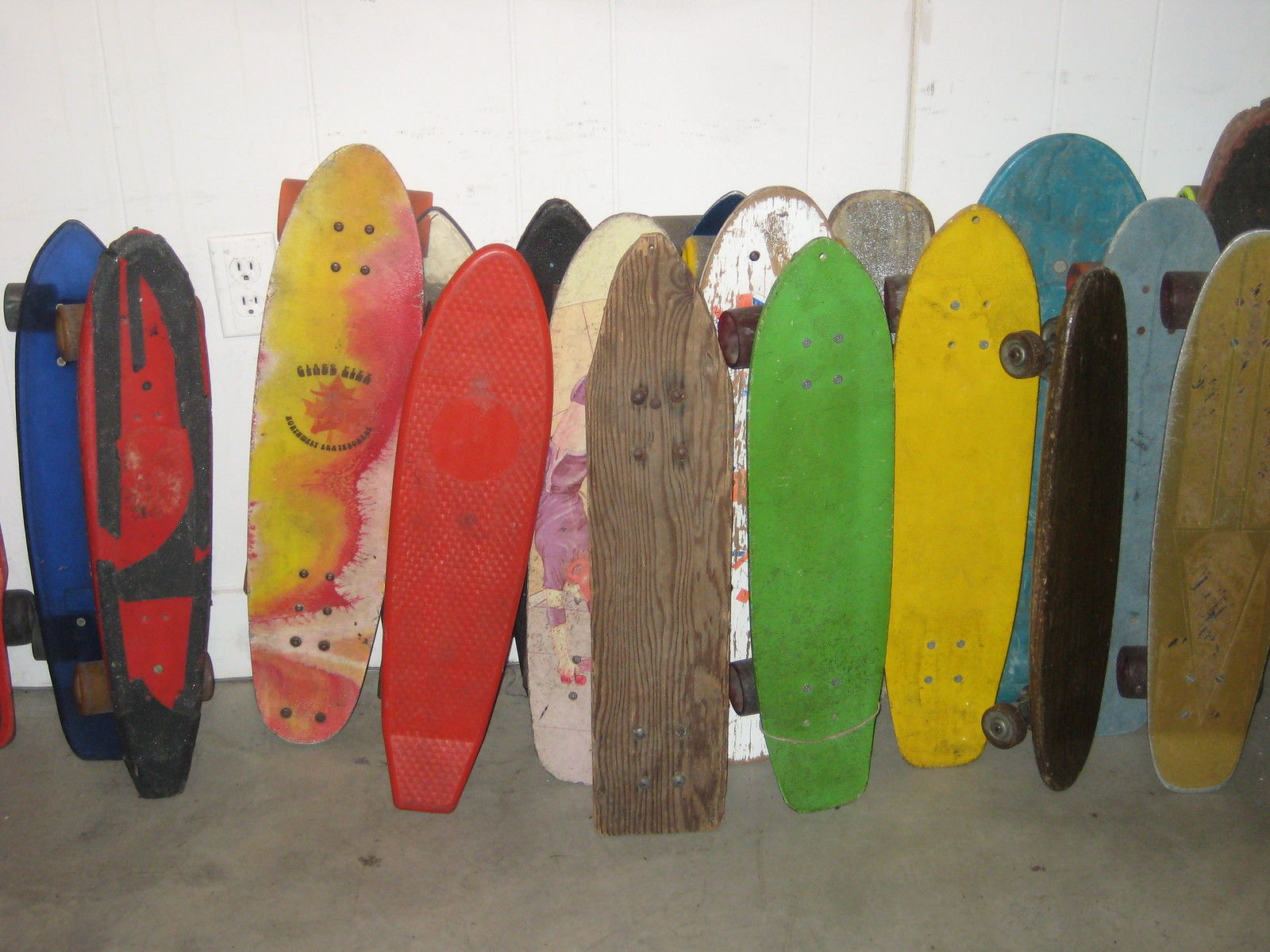The image depicts a collection of mini skateboards leaning against a white wooden wall, which appears chipped and dingy in places. The skateboards, showcasing evident wear and tear, are arranged side-by-side on a concrete floor. They vary greatly in shape and color; some are rounder and others narrow and short. The assortment includes boards in green, yellow, blue, purple, red, orange, and plain wood finishes. Some have faded paint, especially noticeable on the tips, while others are adorned with patterned designs. While most of the skateboards lack wheels and display the holes where the wheels would be attached, a few are fully outfitted with black wheels. The collective display highlights an eclectic mixture of textures and finishes, with some boards sporting a matte color scheme.